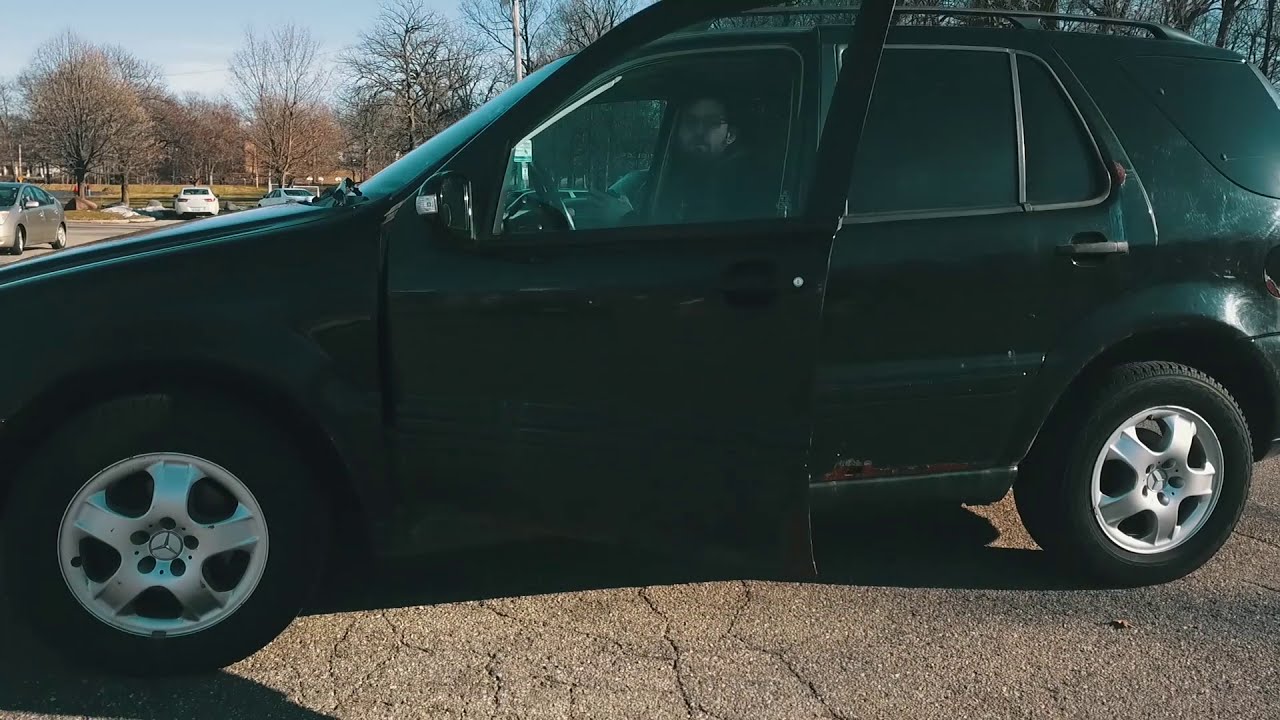This color photograph, taken in landscape orientation, captures a detailed side view of a black four-door SUV parked on a cracked asphalt surface. The SUV features distinctive silver starfish-shaped rims and has noticeable rust at the edge of the open driver's side door. Seated behind the steering wheel is a Caucasian male, likely in his early to mid-30s, sporting glasses and a handlebar mustache and beard, who is looking directly towards the camera. The background reveals a nearly bare winter landscape with leafless trees, faint patches of snow on the grass, and three distant vehicles - two white cars further back and a silver car positioned midway between the black SUV and the white cars - all arranged in a parking lot under a clear light blue sky.